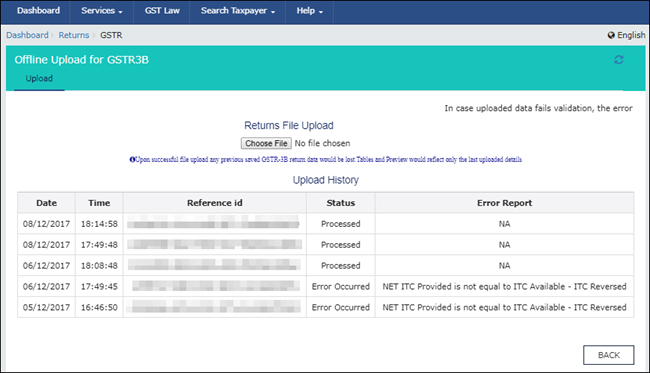The image depicts a detailed dashboard interface for a GST (Goods and Services Tax) application. At the top, there's a dark blue navigation bar with white text displaying options: "Dashboard Services," "GST Law," "Search Taxpayer," and "Help." To the far right of this bar, it is specified that the language is English.

Below the navigation bar, there is a light blue header labeled "Dashboard Returns" and a black "GSTR" heading. Following this is a teal field with the white text "Offline Upload for GSTR 3B," highlighting an active "Upload" tab and a refresh icon on its right.

Further down on the main white section, there is a notice saying, "In Case Uploaded Data is False, Validation, the Error." Centered below this in a line of text is "Returns File Upload," followed by a "Choose File" selection button with no file chosen at the moment. There is some unreadable instructional text in blue beneath it.

The bottom section features a database grid with columns titled in bold: "Date," "Time," "Reference ID," "Status," and "Error Report." The date entries show "8-12-2017" for the first two rows, "6-12-2017" for the next two, and "5-12-2017" for the last row. Corresponding time entries include "18-14-58," "17-49-48," "18-08-48," "17-49-45," and "16-46-50" respectively. The status for the first three entries is "Processed," while the last two show "Error Occurred." The error reports detail "Non-Available" for the first three entries, and "NET ITC Providers Not Equal to ITC Available, ITC Reversed" for the last two entries.

A "Back" button is positioned in the lower right corner of the dashboard.